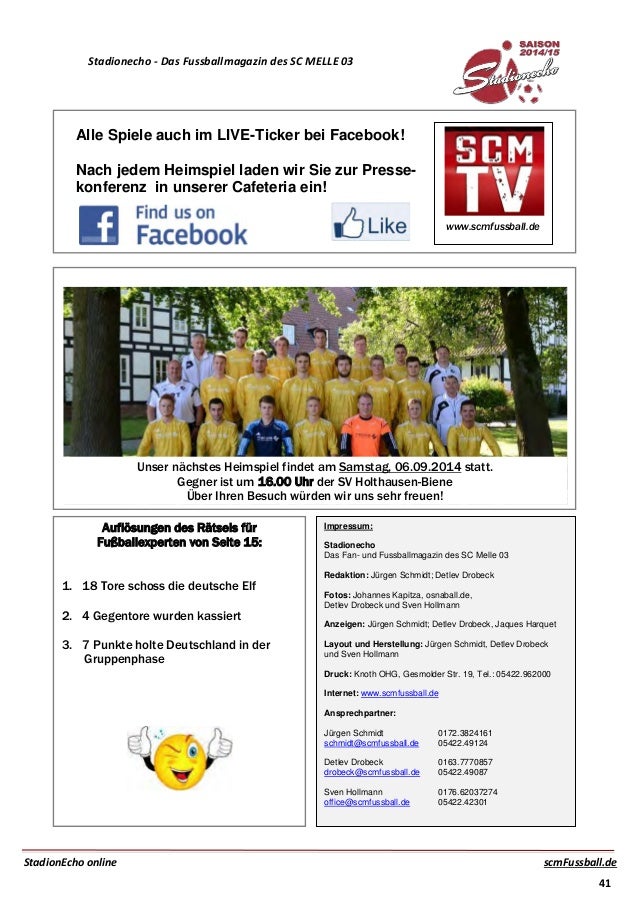This image is a cropped portion of a web page or advertisement, written in what might be German, with the year 2014-2015 displayed prominently in the upper right corner. The site apparently belongs to SCMTV (SCM TV), with references to "Find us on Facebook" and a Facebook like button also visible. The main feature of the image is a photograph depicting a large group of young adults, possibly students, standing in front of a building flanked by two trees. There are about 21 to 30 individuals arranged in rows, with most of them dressed in long-sleeve yellow shirts adorned with white text that’s unreadable. Additionally, the page includes various graphics and several colors, including white, black, red, yellow, light blue, and gray. The text appears to be informational, containing contact details, dates, and possibly a schedule below the photograph. The overall composition and content suggest that this is an advertisement or informational flyer.